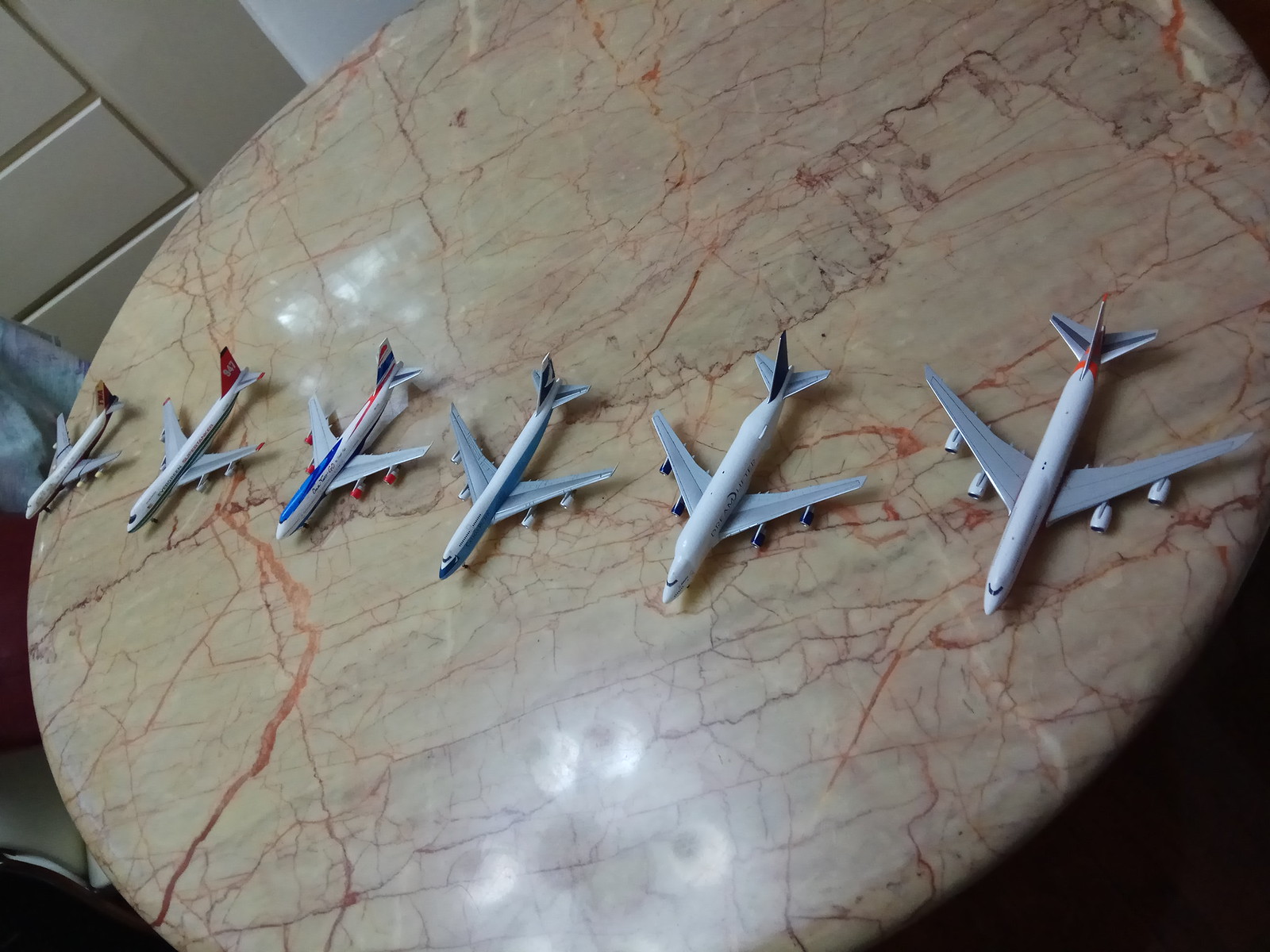The image depicts a detailed photograph of a marble table adorned with six model airplanes, arranged in a horizontal line across the center of the surface. The table itself is an elegant light beige, almost ivory in color, with intricate veining in shades of red, maroon, and dark brown that resemble scribbles. Above the table, the reflection of multiple light bulbs hints at a chandelier overhead.

The airplanes vary in size, with the largest positioned on the right and the smallest on the left. These models predominantly feature white exteriors accented by touches of red, blue, and a little bit of yellow. Specifically, the largest plane on the far right is distinguished by silver and blue markings on its tail, while the smallest one on the far left appears to have some yellow on its tail. Each plane displays intricate details: the second plane from the right has a black tail, the third showcases light blue on its lower half, and the fourth includes a blue stripe and red accents. The overall scene combines the sleek design of the airplanes with the intricate beauty of the marble surface, creating a visually rich and complex composition.